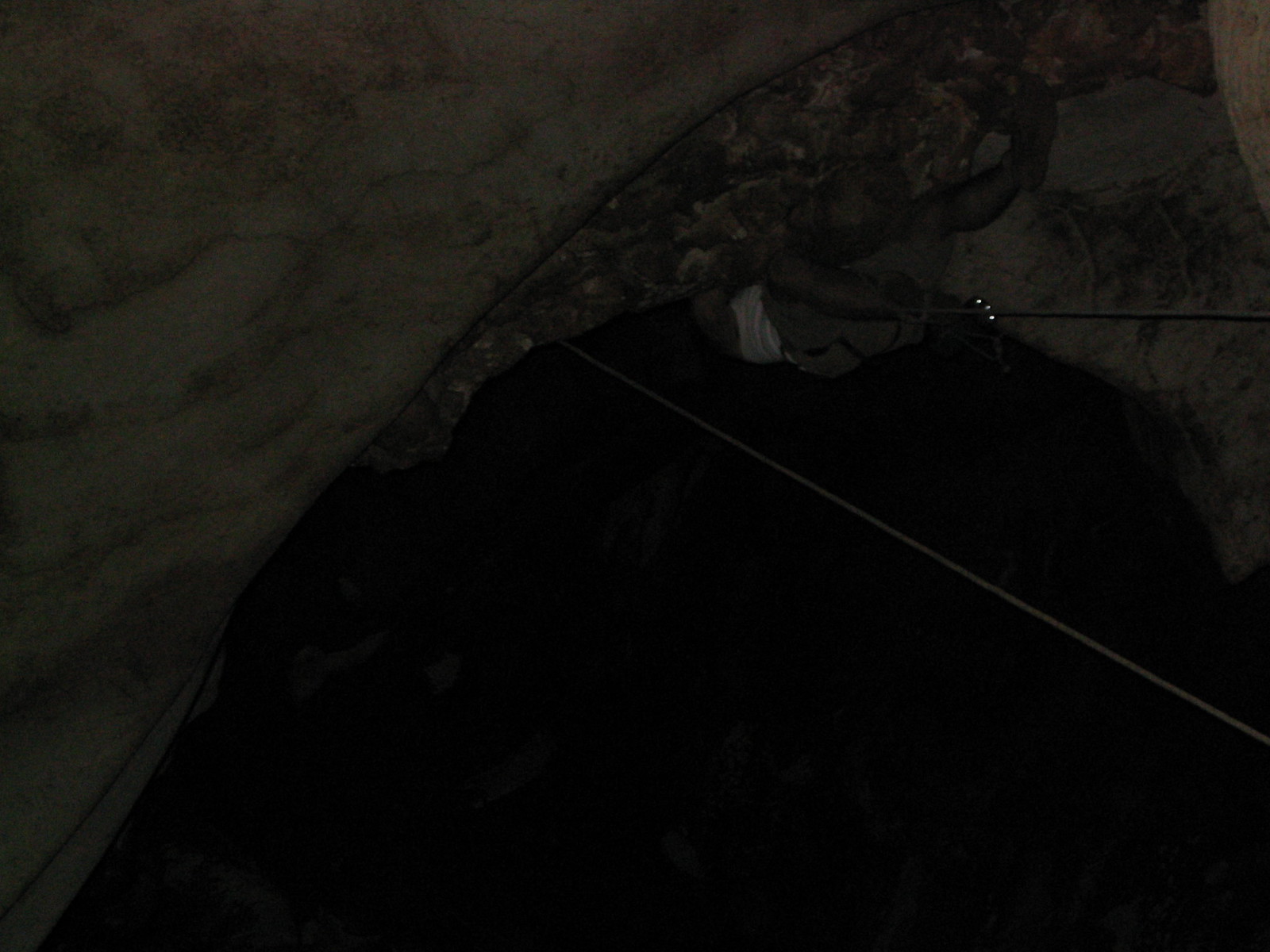In this very dark, nighttime photograph, a man wearing a white tank top and shorts can be seen rappelling down ropes into what appears to be a cave or a natural rock archway. The image is almost completely black at the bottom, with the cave entrance forming a wide, vertical, rectangular shape that arches from the left to the right side of the picture. Two tight ropes, matching the grayish-black color of the rocky arch, extend from the top of the image, angling diagonally downward. The man is positioned on one of these ropes, climbing down from the arched stone structure at the top left. His head is obscured by the rocks, making it challenging to discern his features. The overall scene is hard to make out due to the darkness, but it captures the adventurous activity of rappelling or spelunking at night.